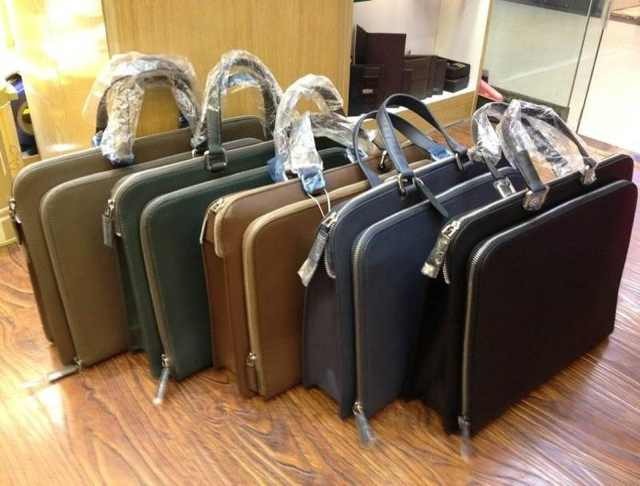This image appears to be taken in an interior setting, likely a store or a private office, featuring a collection of suitcases and briefcases displayed on a medium-dark oak wood floor. The suitcases, five in total, are arranged in a diagonal line from right to left, allowing a clear view of each. The color of the briefcases progresses from black on the far right, followed by blue, tan brown, green, and beige. Each briefcase handle is wrapped in plastic, suggesting they may be recently purchased or intended for resale.

In the upper right corner of the image, a mirrored sliding glass door is visible, reflecting parts of the room and hinting at additional suitcases or possibly other items on a shelf. This contributes to the perception of a store-like environment or a well-organized office. The contrast between the warm tones of the wooden floor and the neutral and darker shades of the leather suitcases creates a visually appealing composition.